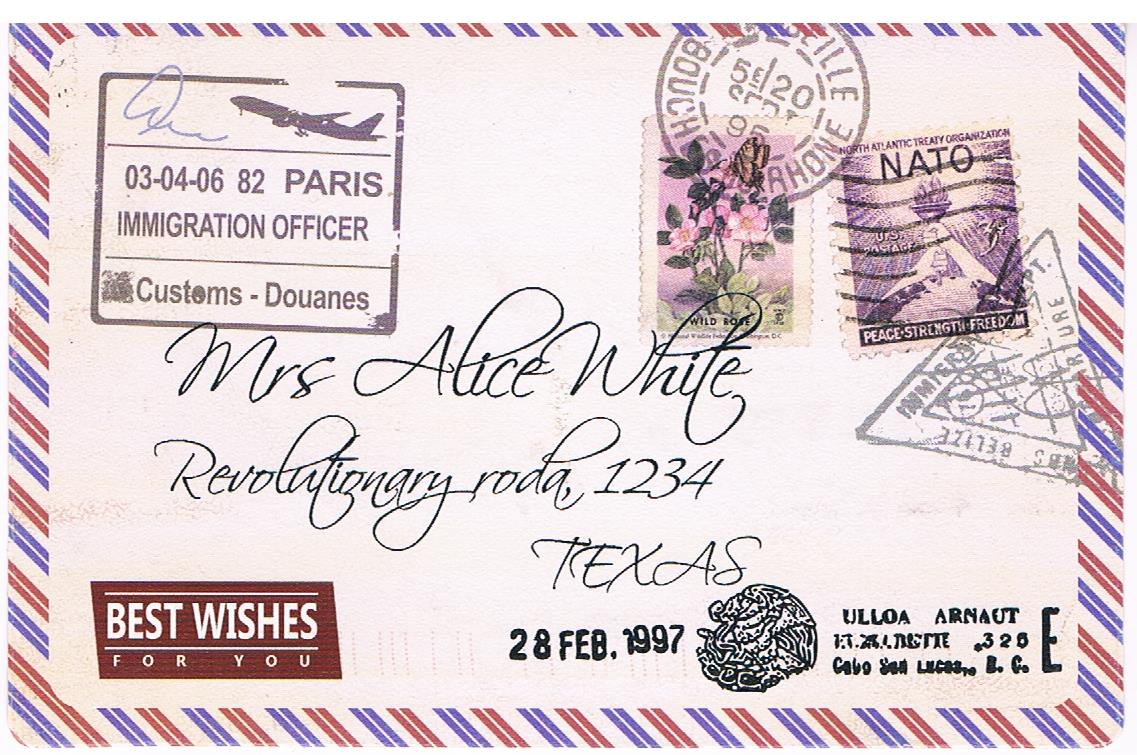This image shows a detailed postcard, which occupies the entire frame. The postcard features a distinctive red, white, and blue striped border reminiscent of a barbershop pole, suggesting it's intended as airmail. The central focus is an address label directed to Mrs. Alice White, Revolutionary Road, 1234 Texas. Adorned with various stamps and postal marks, there's a notable ink stamp at the top that reads "Immigration Officer Customs Mrs. Alice White," alongside phrases like "Best Wishes for You" in the bottom left. The upper section contains multiple stamps, including circular, triangular, and traditional postage stamps depicting an airplane, NATO, flowers, and a date mark of 28 February 1997. The intricate design includes overlapping elements, with some text rendered difficult to read but contributing to the rich, layered aesthetic of this fascinating piece of mailed history.